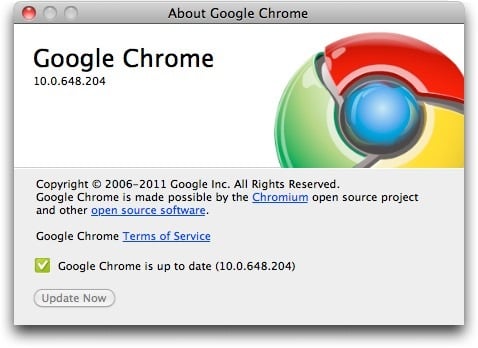In this image, we see a screenshot featuring a primarily gray and white color scheme. At the top, there's a dark gray header with three circles on the upper left-hand side. The first circle is shaded in red, giving it a marbled appearance. Below the header, on the right side of the screen, the Google Chrome icon is displayed in a digitally rendered, three-dimensional rounded design against a solid white background. To the left of the icon, in large bold text, it reads "Google Chrome 10.0.648.204". On the lower half of the image, set against a light gray background, there is a copyright notice stating "© 2006 - 2011 Google Inc. All rights reserved". It also mentions that "Google Chrome is made possible by the Chromium open source project and other open source software," with "open source software" highlighted as a clickable blue link.